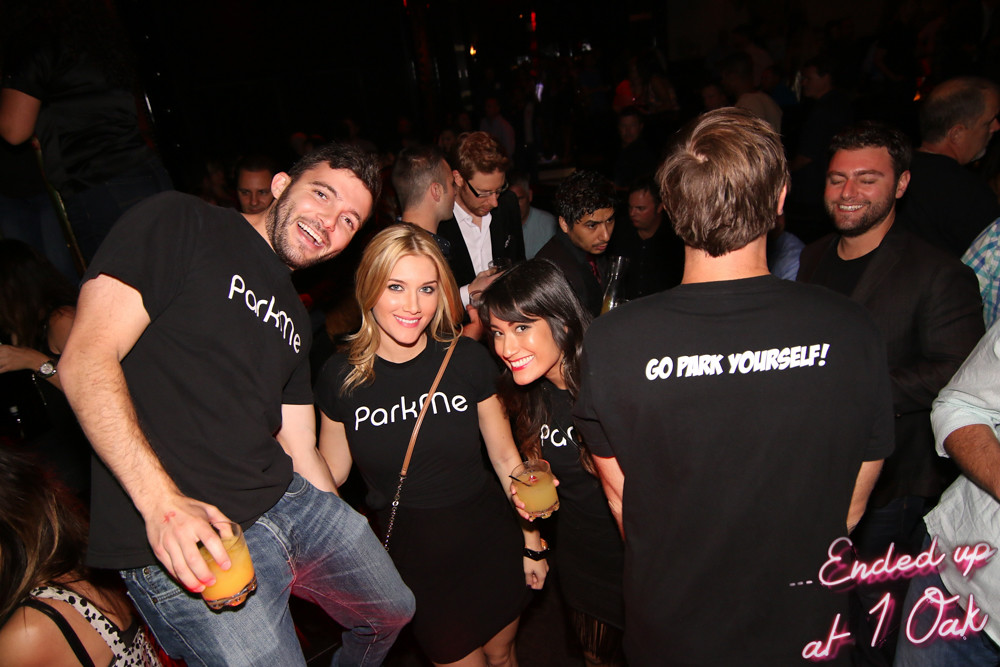In this vibrant, indoor nightclub scene set at night, a group of people are enjoying their time at what appears to be One Oak, as indicated by the purple neon text "Ended up at One Oak" in the bottom right corner. The foreground prominently features a white man with short brown hair, wearing a black short-sleeved t-shirt emblazoned with "Park Me" and blue jeans. He holds a glass containing an orange liquid in his right hand.

Next to him, on his right, stands a blonde woman who also sports a black "Park Me" t-shirt and is smiling warmly. She carries a crossover purse and has her arms down by her side. Beside her is an Asian woman wearing bright red lipstick, beaming at the camera while holding a similar drink.

To their right, a white man with his back turned to the camera wears a black t-shirt that reads "Go Park Yourself" in white letters. He is engaged in conversation with a man in a black sports jacket, who is looking down and smiling.

In the background, partially visible amidst the darker setting and flashing lights, is a group of people. An Asian man looks downwards, and a white man with glasses dressed in a sports jacket and white shirt also gazes down. A general festive and social atmosphere permeates the scene, with the crowd appearing to enjoy the lively ambiance of the club.